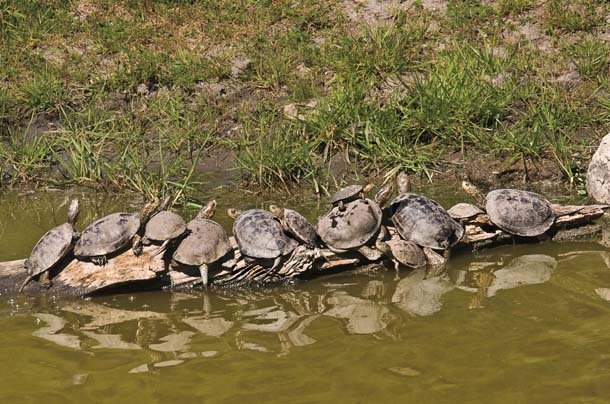The photograph, in landscape orientation, features a serene and natural scene of about a dozen turtles perched on a piece of driftwood at the edge of a shallow, greenish-brown body of water. The driftwood, situated horizontally and slightly tilted towards the bottom left, extends from one side of the image to the other, providing a resting spot for the turtles. Most of the turtles, with their brownish mud-colored and grey shells, are clustered closely together, with some even overlapped on the left side. A small turtle stands out on the right, facing a different direction.

The water beneath the driftwood is shallow and reflective, mirroring the turtles above. The top half of the image reveals a muddy bank of the creek, lush with clusters of long green grass, transitioning to dry, grey soil in the uppermost portion. The detailed representation captures the tranquil coexistence of these creatures within their natural habitat.